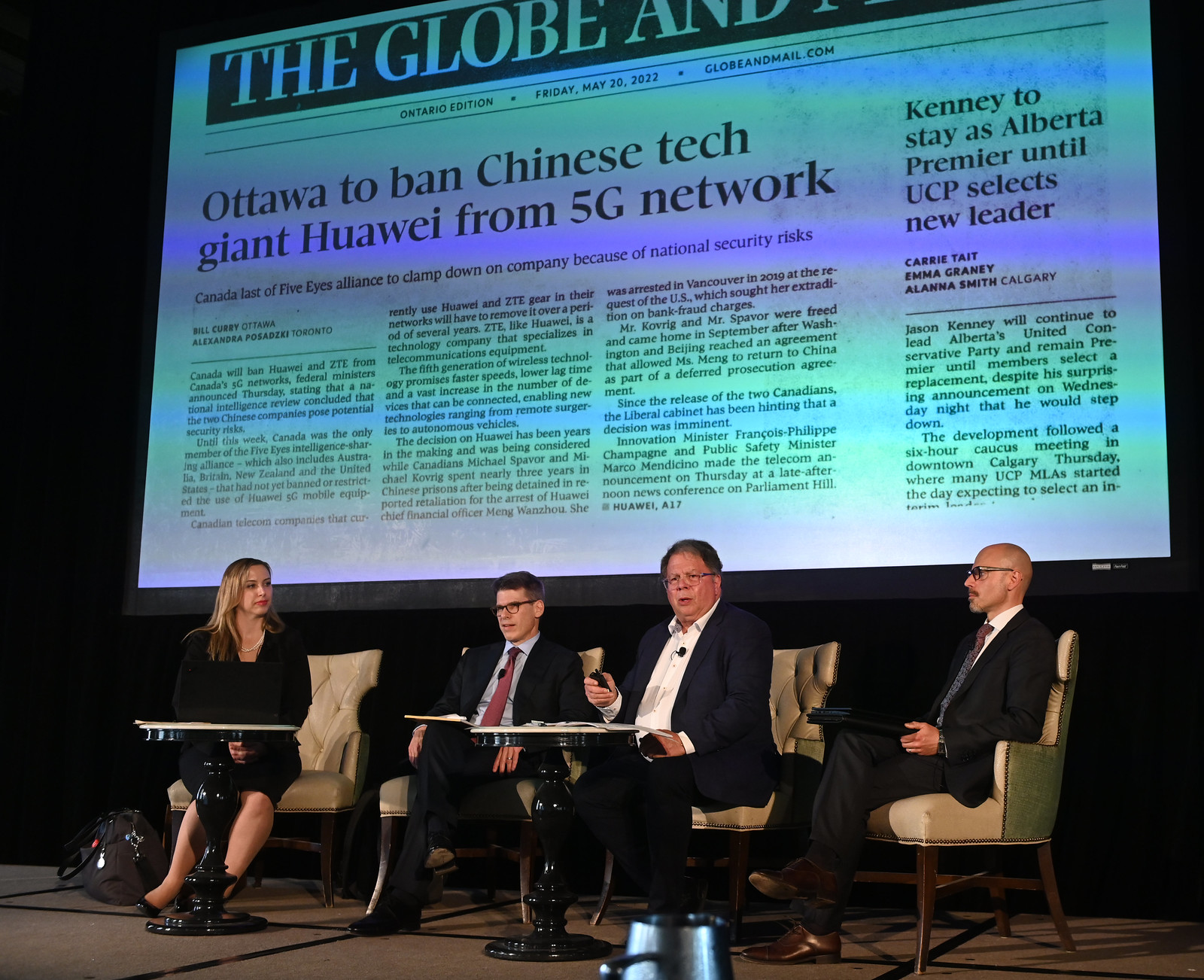The image depicts a formal panel set on a slightly carpeted or hard-floored stage, where four individuals—three men and one woman—are engaged in a presentation or discussion. The men, dressed in suits with one notably without a tie, and the woman, adorned in a black dress with a pearl necklace, are seated on elegant tan leather chairs with wooden legs. In front of them are two tables. The woman has a bag beside her. Behind them, a large projector screen displays headlines from The Globe and Mail, dated Friday, May 20th, 2022, with the prominent articles, "Ottawa to ban Chinese tech giant Huawei from 5G network" and "Kenny to stay as Alberta Premier until UCP selects new leader." The background is draped with a black curtain, giving the setting a professional and focused ambiance. This indoor scene clearly indicates a formal event, such as a symposium or a debate, where the panel is likely addressing questions from an audience. The screen’s image, although partially obscured, emphasizes critical national and political news, adding context to the significance of the panel discussion.